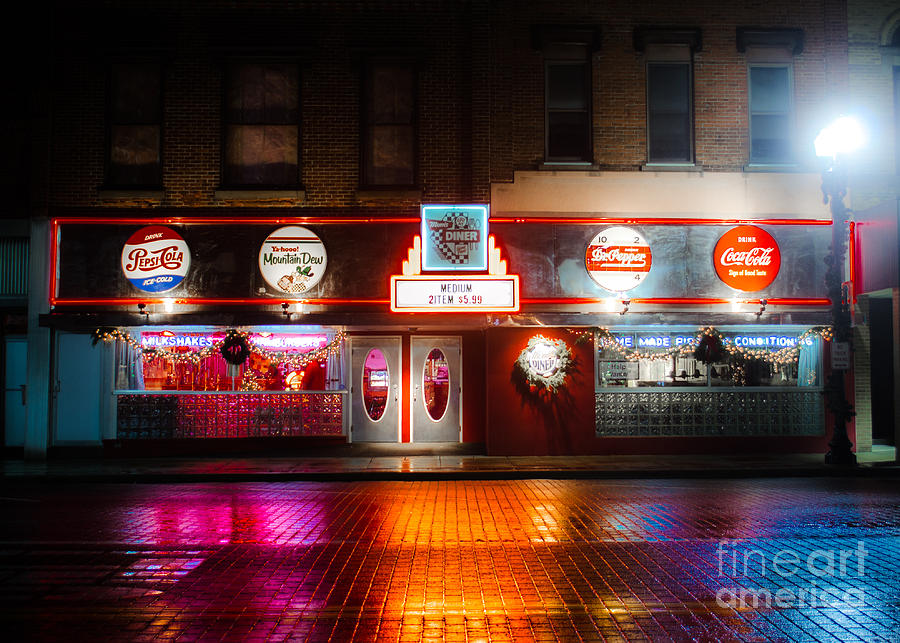The image depicts the vibrant front view of a retro-futuristic American diner at night, brimming with colorful neon signs. Positioned prominently on the building's facade, the neon signs advertise popular sodas: Pepsi, Mountain Dew, Dr. Pepper, and Coca-Cola. Additional signs announce "milkshakes," "hamburgers," and a special offer—medium, two items for $5.99. 

The diner’s holiday spirit is evident with wreaths and garlands adorning its exterior. Two push-in doors are visible, flanked by windows with neon signs that read "milkshakes" and "homemade pies." Street lamps illuminate the scene, adding to the glow of the neon lights that reflect vividly off the wet, cobblestone pavement in front of the building.

A Fine Art America copyright mark is discernible at the bottom right corner of the image, underscoring the artistic quality of the photograph. The overall atmosphere is nostalgic and festive, capturing the essence of a quintessential old-school American diner at night.